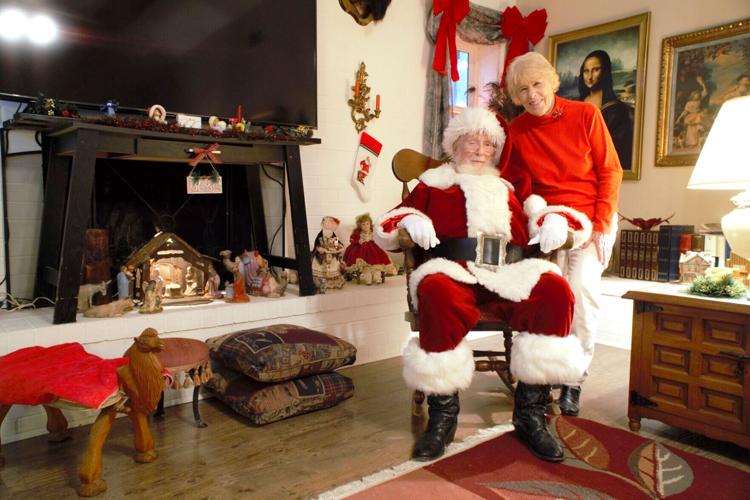The photograph captures an older man dressed as Santa Claus, seated comfortably in a wooden rocking chair. He dons the classic Santa ensemble: black boots with white fur trim, red velvety pants, a matching red velvet jacket with white fur trim along the front, collars, hem, and wrists, white cloth gloves, and a red hat with white fur trim. His long white beard and glasses complement his jolly appearance. Behind him, an older woman—possibly his wife—stands slightly leaning over, smiling warmly. She is wearing white pants, black boots, and a festive red long-sleeve turtleneck sweater. Her blonde hair falls below her ears. They are located in a room with white painted walls and a tannish gray wood floor. The space is decorated for the holidays, featuring Christmas dolls, wreaths, and other seasonal decorations. The right wall displays multiple artworks, including a replica of the Mona Lisa. A large flat-screen TV is mounted above a fireplace, contributing to the cozy, festive atmosphere.